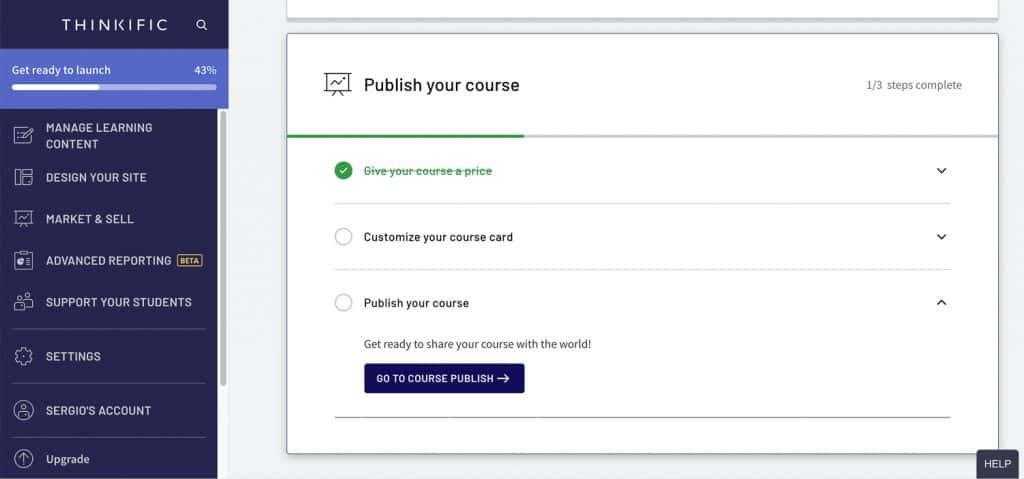The image is divided into two distinct sections: the left and the right.

On the left side, the background transitions from gray to blue vertically. At the top against the blue background, there is white text that reads "Think Griffic". Below it, against a very light blue background, is a magnifying glass icon with the text "Getting ready to launch: 43%". Underneath this text, a status bar is displayed, which is just under half full with white, the remaining portion being gray. Further down, a list of features is presented in white text: "Manage learning content, Design your site, Market and sell, Advanced reporting (Beta)," and more features like "Support your students, Settings, Cirgo’s account, and Upgrade."

On the right side of the image, the background is predominantly gray. There is an empty white box and below it, a larger white box contains black text which reads, "Publish your course: 1/3 steps completed." Under this, a green checkmark is followed by the crossed-out text, "Give your course a price," and a dropdown arrow on the right side. Below this, a gray circle with an arrow pointing down has black text next to it that says, "Customize your course." Further down, another gray circle with an arrow pointing up has black text that reads, "Publish your course." At the very bottom, there's gray text that says, "Get ready to share your course with the world." A dark blue button with white text states, "Go to publish the course" accompanied by an arrow pointing to the right. Finally, against a blue background, the word "HELP" is prominently displayed in white capital letters at the bottom.

This visual layout appears to be part of a tutorial or setup guide for launching an online course.